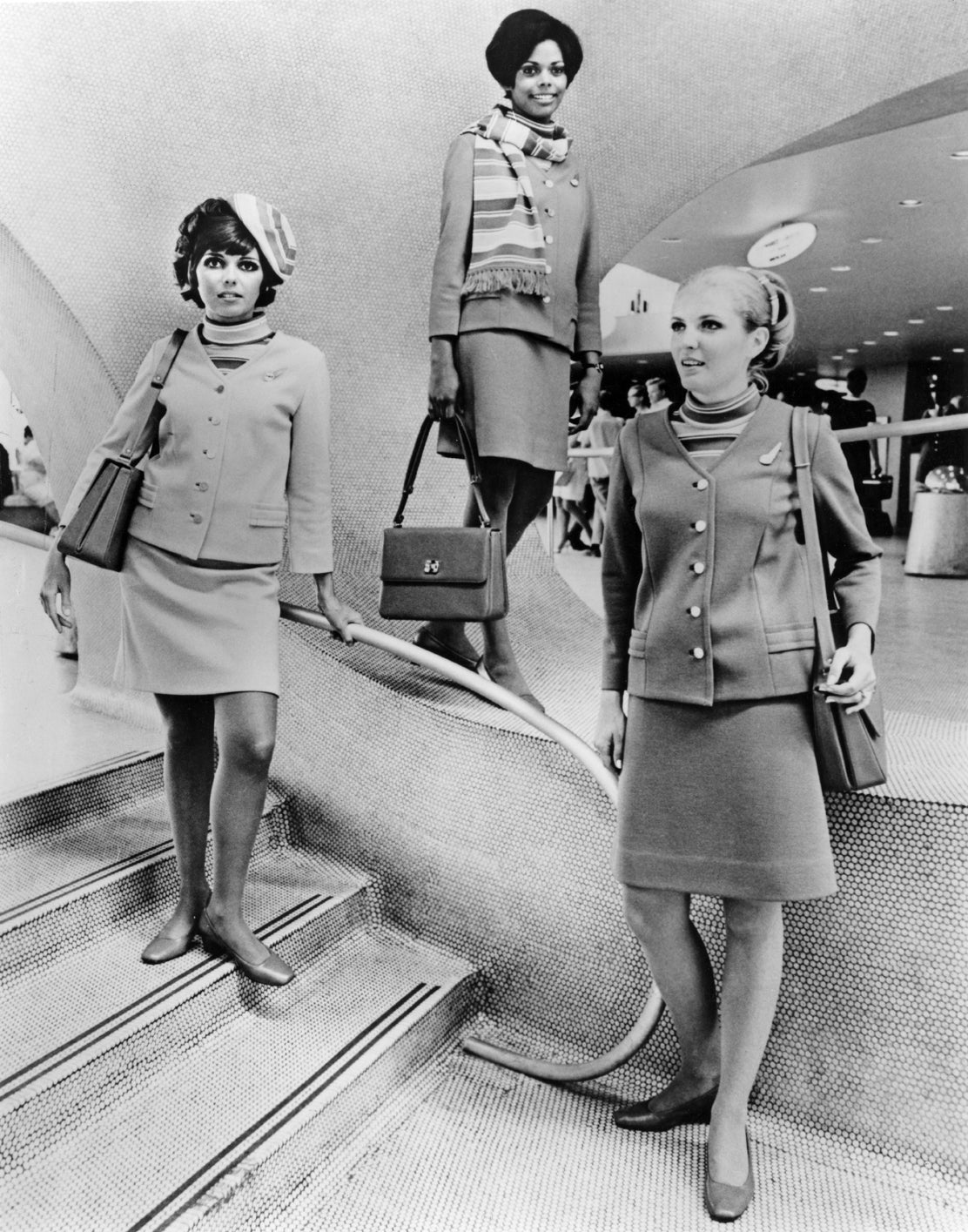This black and white photograph captures a group of airline stewardesses, possibly from an old-school era, posing on a small stairwell with three or four steps, possibly in an airport. The stewardesses are all dressed in identical uniforms, featuring knee-length skirts, jackets, and turtleneck sweaters. Their coordinated outfits include matching purses and shoes, contributing to their uniform appearance. Interestingly, one stewardess stands out with a knitted beanie-style cap worn tilted to the side of her head. Another has a wrap around her neck, adding a slight variation to the cohesive look. They are seen descending the stairs and striking a pose, with their well-coordinated attire highlighting the timeless elegance and uniformity characteristic of airline service staff.